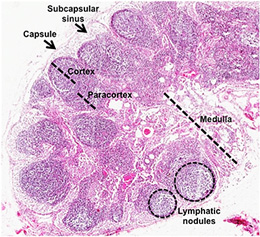The image is a detailed diagram depicting a section of a brain, likely from a human or an animal, viewed against a light gray background. The brain tissue in the diagram is predominantly a light purplish color interspersed with areas of pink and white, creating a floral-like, swirling pattern. Darker fuchsia pink regions are visible, particularly towards the bottom right corner. Several key anatomical features are labeled in clear black text with arrows and dotted lines: "subcapsular sinus" and "capsule" are indicated with solid arrows, while "cortex," "paracortex," "medulla," and "lymphatic nodules" are demarcated with broken lines and dotted circles. The cortex and paracortex run through the upper part of the brain, while the medulla extends along the right-hand side. The lymphatic nodules are highlighted by two concentric circles, one larger than the other. The outer surface of the brain appears encased in a grayish capsule, contrasting with the intricate, colorful internal structures.